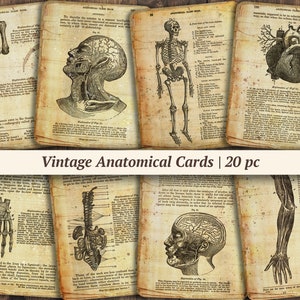The image displays a vintage 20-piece set of anatomical cards, each meticulously illustrating various parts of the human body. The cards, which are yellowed and faded with age, encompass detailed drawings of the head and neck, highlighting different vessels and veins. They also feature comprehensive depictions of the skeleton, labeling bones and joints such as the pelvis, shoulder, and leg bones. Some cards focus on the heart muscle, showcasing its veins, branches, and chambers in great detail. Additional cards cover the anatomy of the arm, labeling its veins, arteries, and hand bones, while others detail the spine, highlighting the various sections and spinal cord. Each card is filled with small print and intricate diagrams, reminiscent of clinical teaching tools from the mid-20th century. The overall collection presents a thorough and educational view of human anatomy.